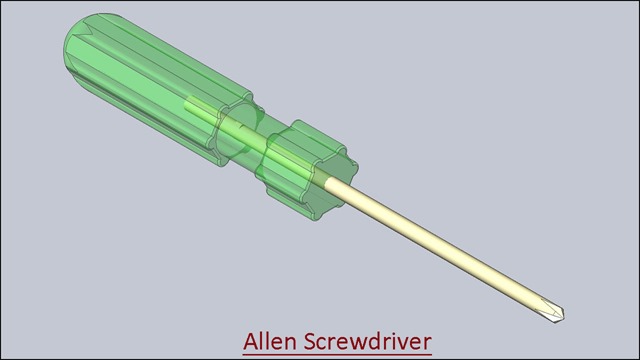This computer-generated image depicts a screwdriver labeled as an "Allen Screwdriver." The entire scene is framed by a thin black border, set against a light gray background. The screwdriver, rendered in a 3D-style graphic, is positioned diagonally with its clear green plastic handle in the top left corner and the beige-colored metal rod extending to the bottom right. The rod ends in a tip shaped like a bunch of diamonds, indicating an unusual design. Below the screwdriver, centrally placed red text reads "Allen Screwdriver," highlighted with an underline. The clean, simple design suggests it might be part of an instructional flash card or similar educational material. No people or additional elements are present in this non-realistic image.